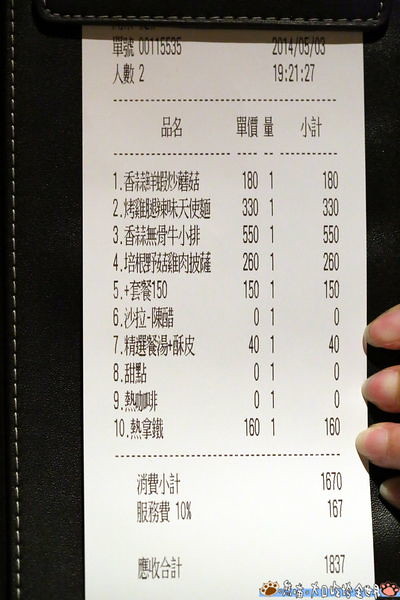The image depicts a white receipt with black text, placed on a leather-like folio and framed by a black border with a dashed, sewing line design along the left and top edges. The receipt is in an East Asian language, likely Chinese. At the top left, there's an ID number "00115535" and to the right, the date "2014/05/03" along with the time "19:21:27". The receipt lists 10 items numbered 1 through 10, each described in Chinese characters. Prices of individual items include 180, 330, 550 (the most expensive), 260, and 160, among others. There are also three items listed at zero cost. Below the item list, it shows subtotals, a 10% tax of 167 units, and a final total of 1837 units.